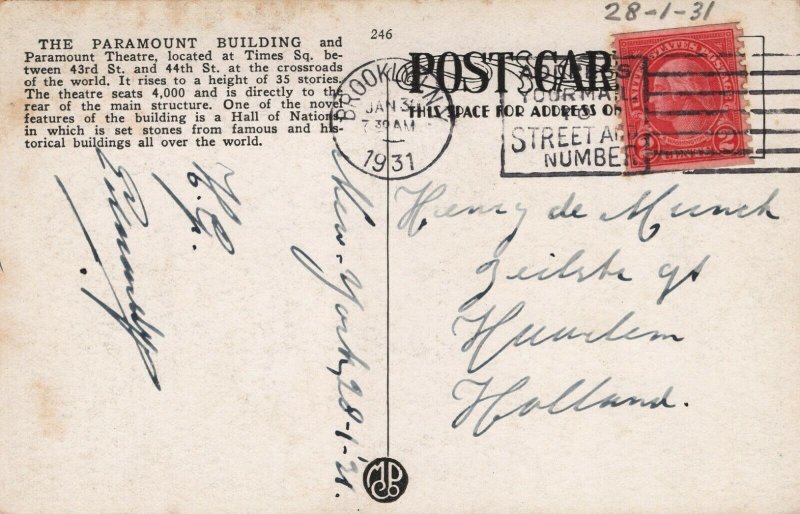This is a close-up of the back of an old postcard from January 30, 1931, sent from a Brooklyn Post Office at 7:30 a.m. The edges of the postcard show visible wear and tear, indicating its age. In the top right corner is a bright red 2-cent stamp featuring George Washington, and alongside it, various ink stamp markings, including one that reads "Brooklyn."

The postcard’s text is divided into two sides. On the left, it describes the Paramount Building and Paramount Theater, located at Times Square between 43rd Street and 44th Street, and rising to a height of 35 stories. The theater seats 4,000 people and is directly behind the main entrance. This text includes details of the building's significance and historical context.

On the right side, there's a handwritten message that begins with a casual greeting, "Hi, how are you doing?" and continues with the name Henry D. Munch, and the address Gilchrist Court. The colors of the postcard include red, beige, and black, enhancing its vintage look.